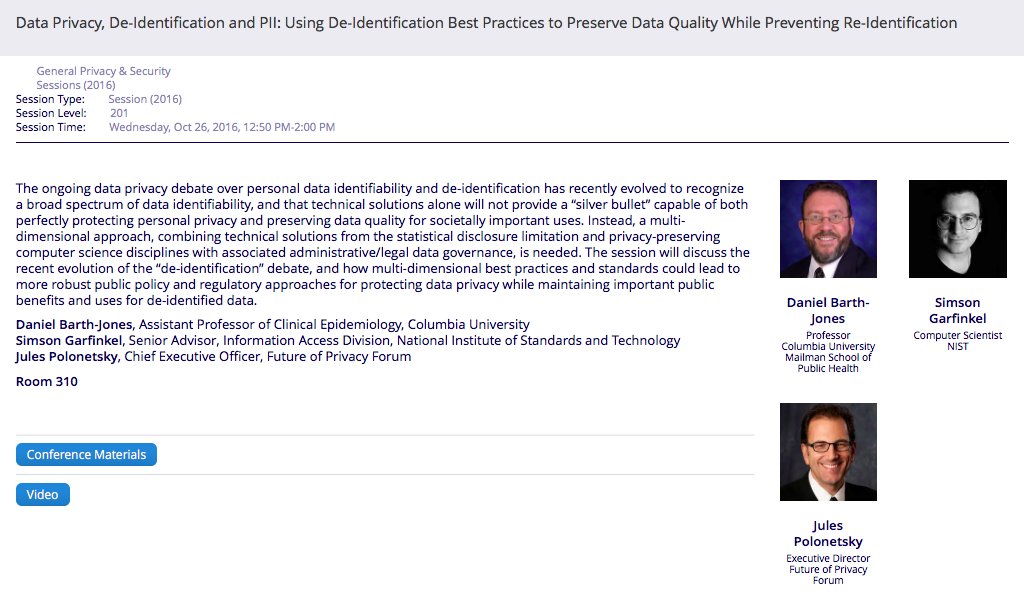The image is a detailed session description box featuring a light gray header with black text. The header reads: "Data Privacy, De-identification, and PII: Using De-identification Best Practices to Preserve Data Quality While Preventing Re-identification." Below the header, additional session details are meticulously listed:

- **Session Title**: General Privacy and Security Session 2016
- **Session Type**: Session 2016
- **Session Level**: 201
- **Session Time**: Wednesday, October 26, 2016, from 12:50 p.m. to 2:00 p.m.

The text indicates that the session focuses on the evolving debate over the identifiability of personal data and the methodologies for de-identification. It acknowledges that a purely technical solution is insufficient to perfectly balance personal identification protection with data quality preservation. Instead, it advocates for a multidimensional approach that integrates technical solutions from statistical disclosure limitation and privacy-preserving computer science with associated administrative and legal data governance measures. This comprehensive method aims to address the complexities of maintaining data privacy in a manner beneficial for societally important uses.